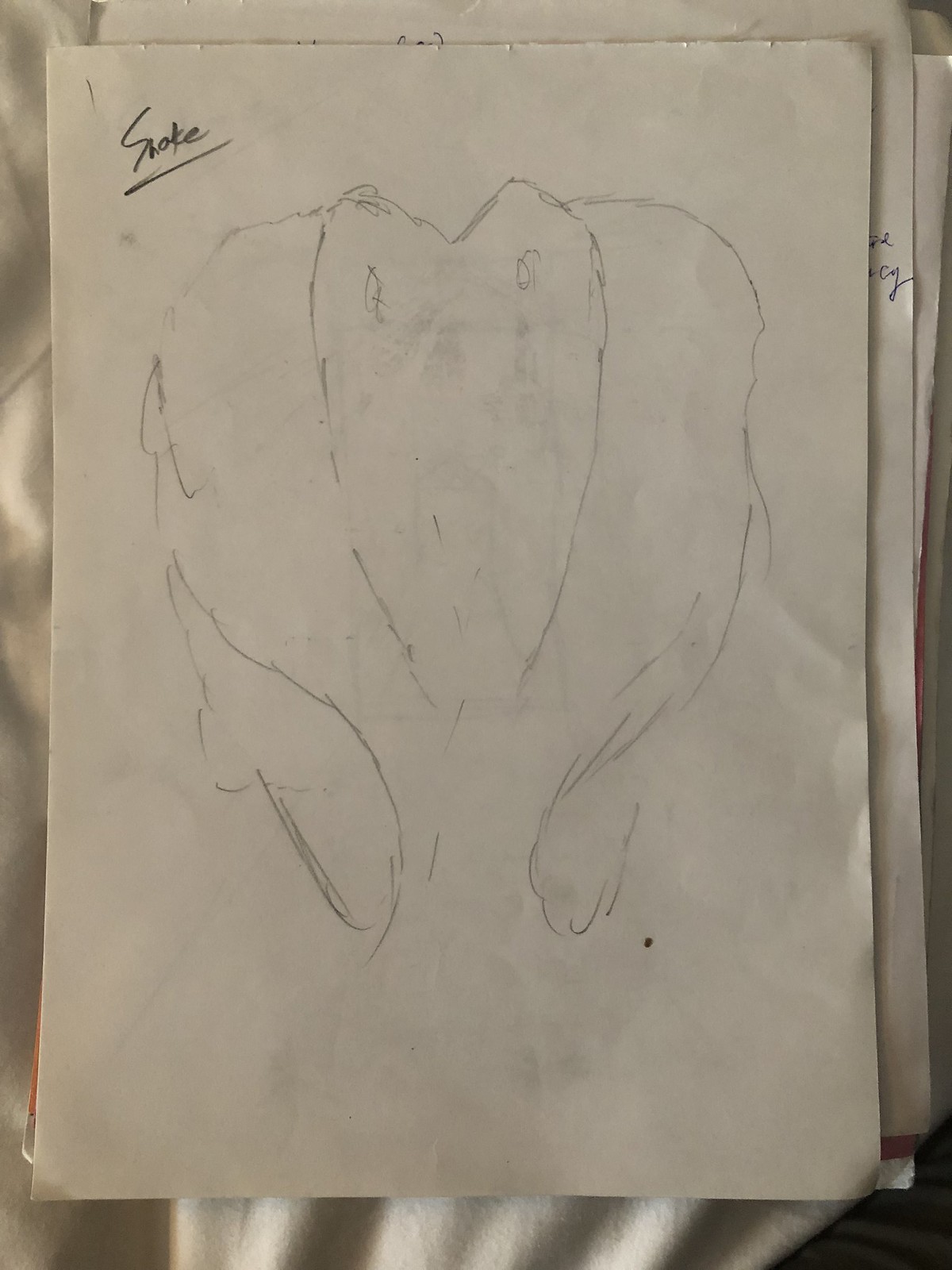This image features a detailed pencil sketch on a white sheet of paper, which rests atop a stack of similar white papers. The paper directly beneath shows hints of cursive writing in black ink. The sketch itself is intriguing and abstract, depicting a heart-shaped center with two eye-like shapes enclosed within it. Extending symmetrically from either side of the heart are forms that resemble a body, narrowing toward the bottom and giving the sketch a cohesive yet enigmatic appearance. The stack of papers is placed on a white cloth, which in turn is draped over a brown wooden table, adding a textured and layered background to the composition.